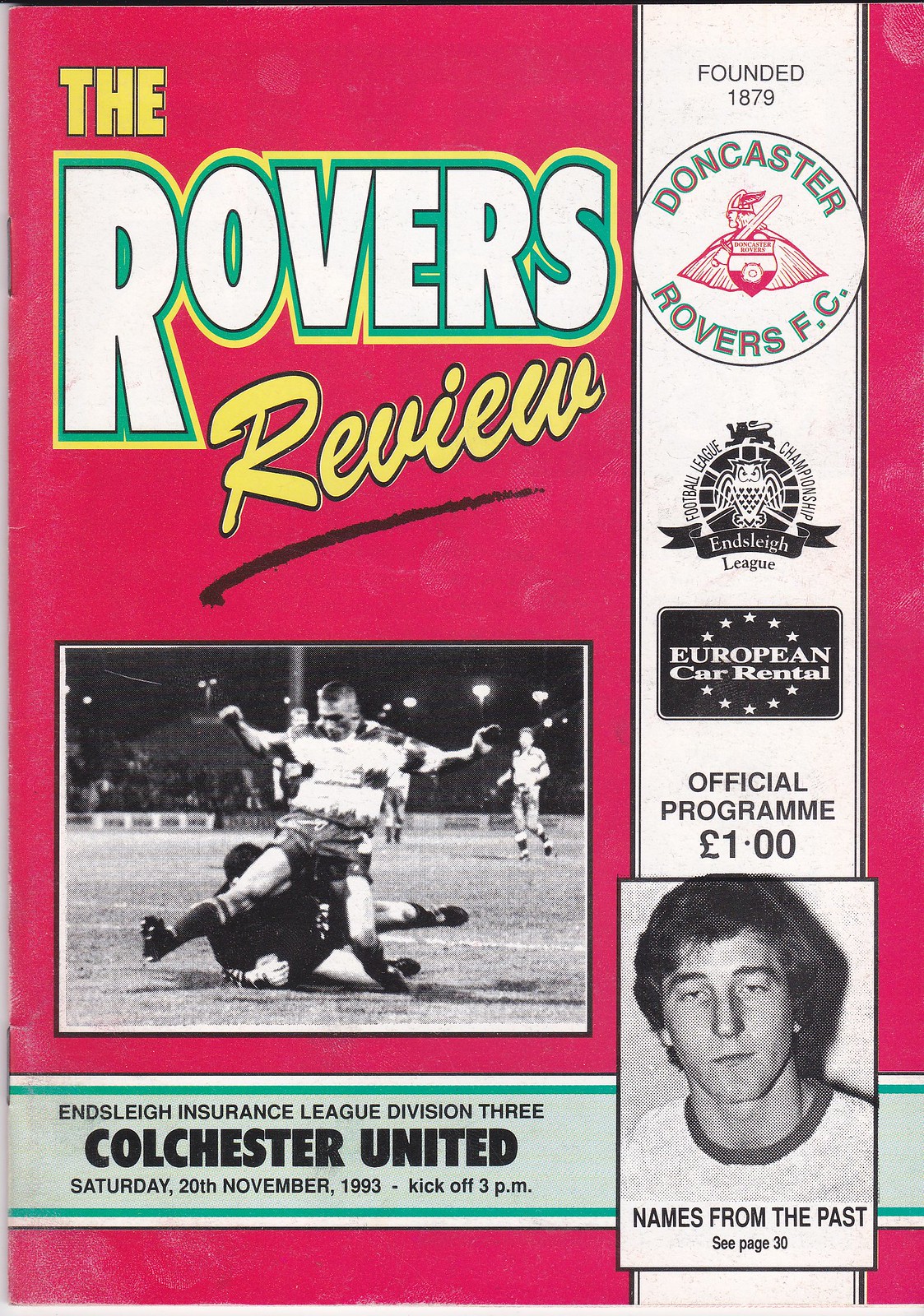The cover of the vintage British soccer magazine "The Rover's Review" features a striking design on a pink background. In the upper left corner, the title "The Rover's Review" is prominently displayed, with "The" and "Review" in cursive yellow font, and "Rovers" in white font bordered with green and yellow. Beneath the title, there is a black and white photograph capturing a dramatic on-field moment where one footballer in a black jersey appears to be falling onto another player in a white jersey, both seemingly engaged in a physical clash on the soccer field.

Below the photo, a green rectangular strip reads: "Ensley Insurance League Division III, Colchester United, Saturday, 20th November, 1993, kickoff 3 p.m." Along the right edge of the cover, a white vertical strip lists important details beginning with "Founded 1879," followed by a circular logo of Doncaster Rovers FC, which includes an emblem of a Viking warrior.

Further down, there is another emblem, this one in black, featuring various elements including a lion, an owl, and the text "Football League Championship" with "Ensley League" inscribed on a ribbon. Directly beneath this is a black rectangular box with "European Car Rental" flanked by stars.

At the bottom, the cover states "Official Program, £1" and includes a small black and white photograph of a young, clean-shaven man with tousled hair, wearing a white t-shirt with black borders. Below this image, the caption reads, "Names from the past, see page 30."